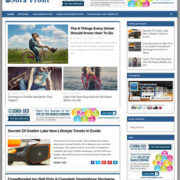The image captures a screenshot of a visually engaging website. At the top of the webpage, a lively photograph features a boy riding a bike while a girl perches on the handlebars, adding a whimsical touch to the scene. Below this, a second image partly reveals the midsection and slightly tilted head of a person, suggesting a candid, introspective moment.

Further down the page, another compelling image displays a girl dressed in a plaid long-sleeve shirt, standing in front of what appears to be a beach. She is holding a camera with both hands, aiming to capture a precise photograph, suggesting a moment of focused creativity.

Adding vibrant splashes of color to the layout are three clusters of balloons in shades of yellow, pink, green, and teal. One cluster is partially visible in the top right-hand corner, slightly cropped by the edge of the image. Another group of balloons is situated in the lower right-hand corner, while the final cluster appears more centrally located but towards the bottom of the page, providing a cheerful, scattered effect throughout the design. The webpage also contains various paragraphs of text, enriching the visual storytelling with informative content.